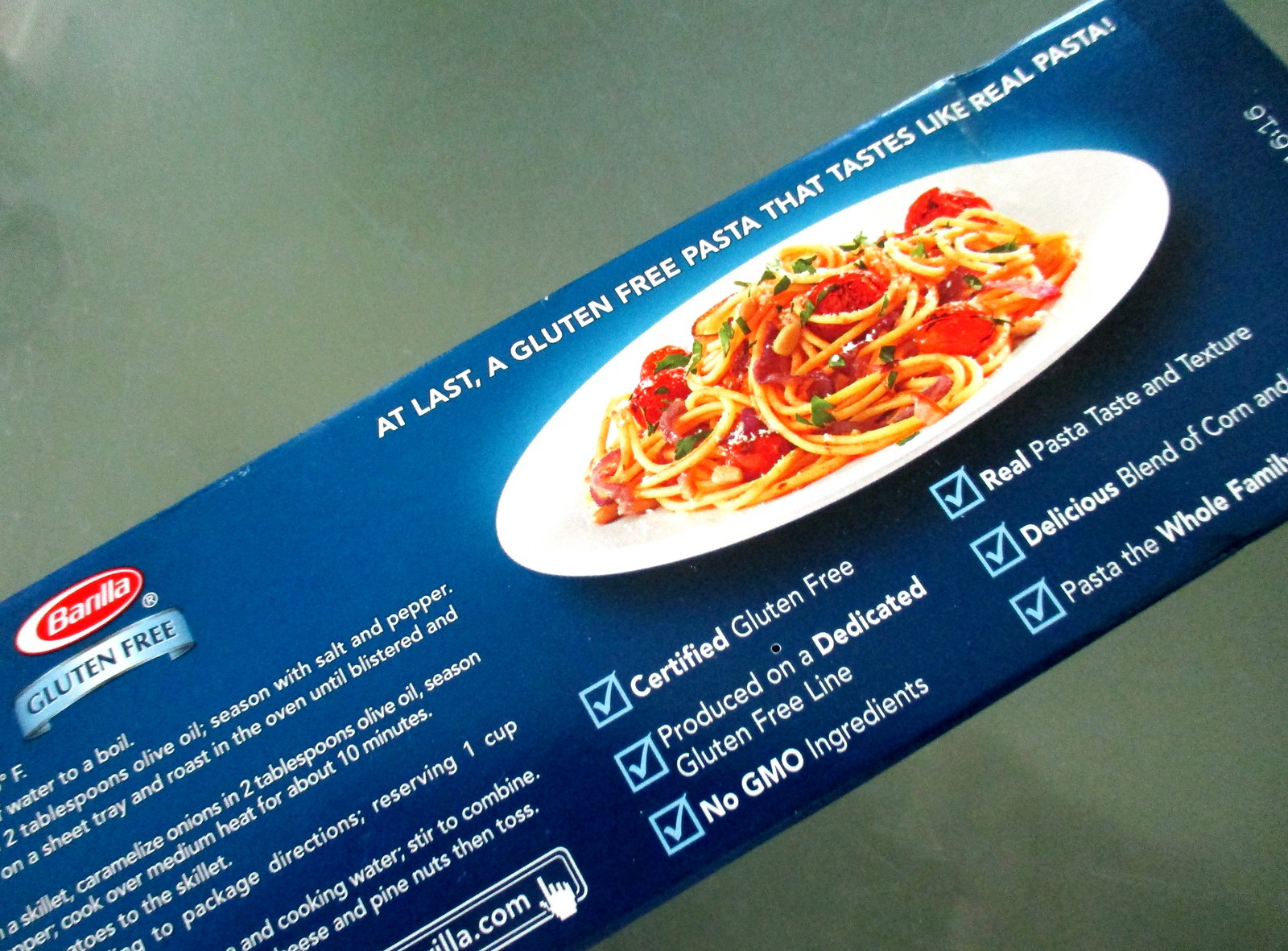This image displays the partial back of a blue box of Barilla gluten-free spaghetti, set against a black background. Dominating the right side of the box is a photograph of cooked spaghetti served on a white plate, garnished with tomato sauce, parsley, and possibly pepperoni. Above the plate, in white font, is the text, "At last, a gluten-free pasta that tastes like real pasta." Below the plate, more product details are provided, including a checklist with text in a blue box that confirms the pasta is certified gluten-free, produced on a dedicated gluten-free line, and contains no GMO ingredients. To the left, additional text highlights the pasta's authentic taste and texture, along with the benefits for the whole family, though this section is partially obscured. Further left, the Barilla logo is visible with a red marker indicating "gluten-free." The left side also features cooking instructions, discussing steps such as bringing water to a boil and using olive oil, although some instructions and a potential website link are cut off.